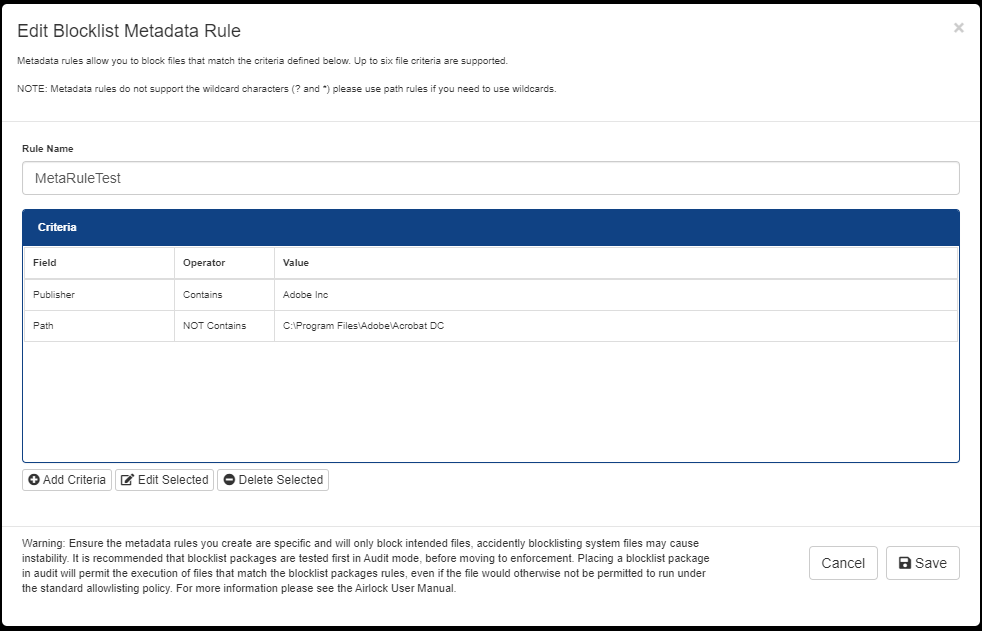This is a highly detailed screenshot depicting the "Edit Block List Metadata Rule" interface.

In the upper left-hand corner, there's a close icon designed to exit the interface, directly opposite of which in the upper right corner, another close icon is crossed out. Beneath this header, textual instructions state: "Metadata Rules allow you to block files that match the criteria defined below. Up to six file criteria are supported. Note, Metadata Rules do not support the use of wildcard characters. Please use path rules if you need to use wildcards."

Continuing downwards, there is a "Rule name" field labeled "Meta Rule Test," formatted in camel case with capital letters "M," "R," and "T." The section below features a blue header labeled "Criteria," which comprises three columns titled "Field," "Operator," and "Value," each in bold font and separated by grid lines.

Under the columns, the first row of criteria consists of "Publisher" under Field and "Contains" under Operator, with "Adobe Inc." listed under Value. The second row has "Path" under Field, "Not Contains" under Operator, and "C:\Program Files\Adobe\Adobe DC" listed under Value. This entire criteria section is displayed within a thin blue-bordered white field.

Below this criteria area, three buttons are aligned horizontally: "Add Criteria," "Edit Selected," and "Delete Selected."

Towards the bottom of the interface, detailed warning lists are present, providing additional context and warnings. Finally, in the lower right-hand corner, there are "Cancel" and "Save" buttons. The "Save" button is distinguished by a floppy disk icon next to it, reinforcing its function to save the changes made.